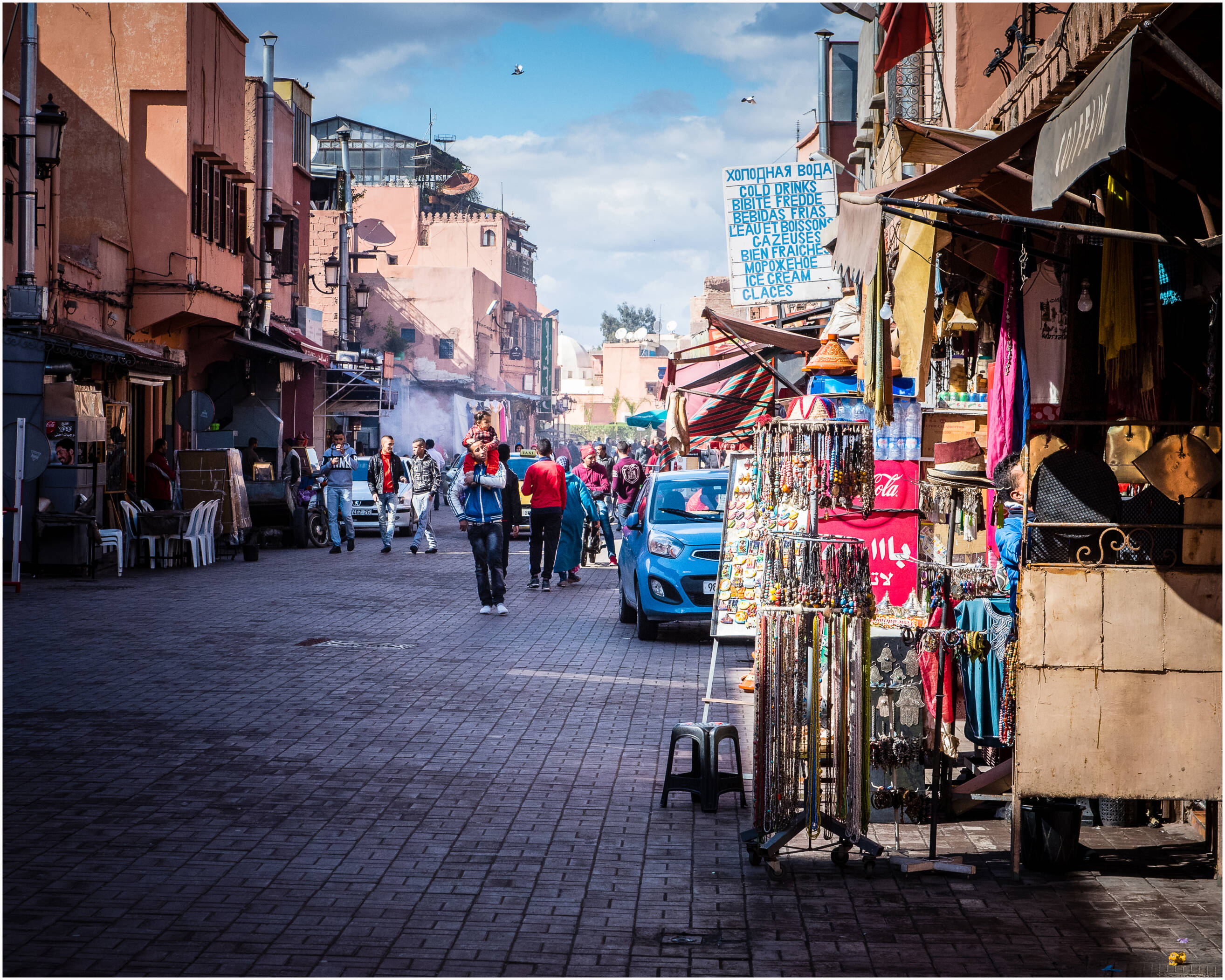The image captures a lively street scene in what appears to be a town center in a possibly Spanish-speaking or third-world community. The road, paved with bricks, is flanked by peach-colored buildings and small shops adorned with overhangs. A vendor's table with white plastic chairs stands at ground level, while various street vendors sell handmade clothes and jewelry. A mix of compact cars and taxis is parked along the sides. A notable detail on the far left is a person carrying a child on their shoulders, adding a touch of warmth to the bustling atmosphere. The blue sky above is dotted with white and gray clouds, and a sign indicating "ice cream, cold drinks" in multiple languages, including what seems like Russian, French, and English, hints at a diverse cultural presence. The street is filled with people, predominantly young men, adding to the vibrant, communal feel of the scene.